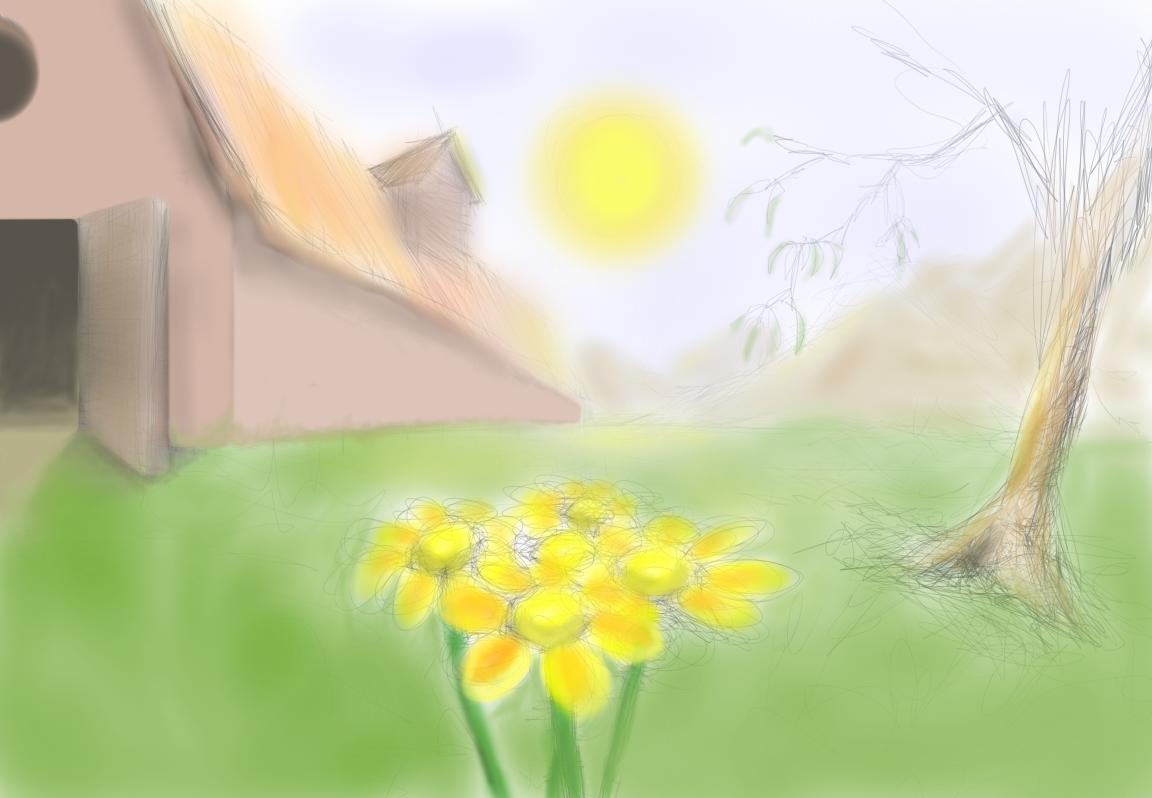This watercolor painting captures a serene rural scene dominated by a large, rustic barn situated at the center. The barn's door is slightly ajar, revealing a dark interior hidden from view. In the foreground, a lush green field dotted with delicate daisy-like flowers, featuring vibrant yellow petals and slender green stems, draws the eye. These flowers serve as a primary focal point, standing proudly in the middle of the composition. Adjacent to the barn, a sparse willow tree, adorned with only a few leaves and bare branches, adds an element of natural elegance. Above the scene, the sun shines brightly, depicted as a well-shaded yellow sphere, providing a beautiful contrast to the predominantly bluish-gray sky filled with soft, billowy clouds, suggesting a mildly overcast day. The painting skillfully balances these elements, creating a tranquil and picturesque countryside atmosphere.